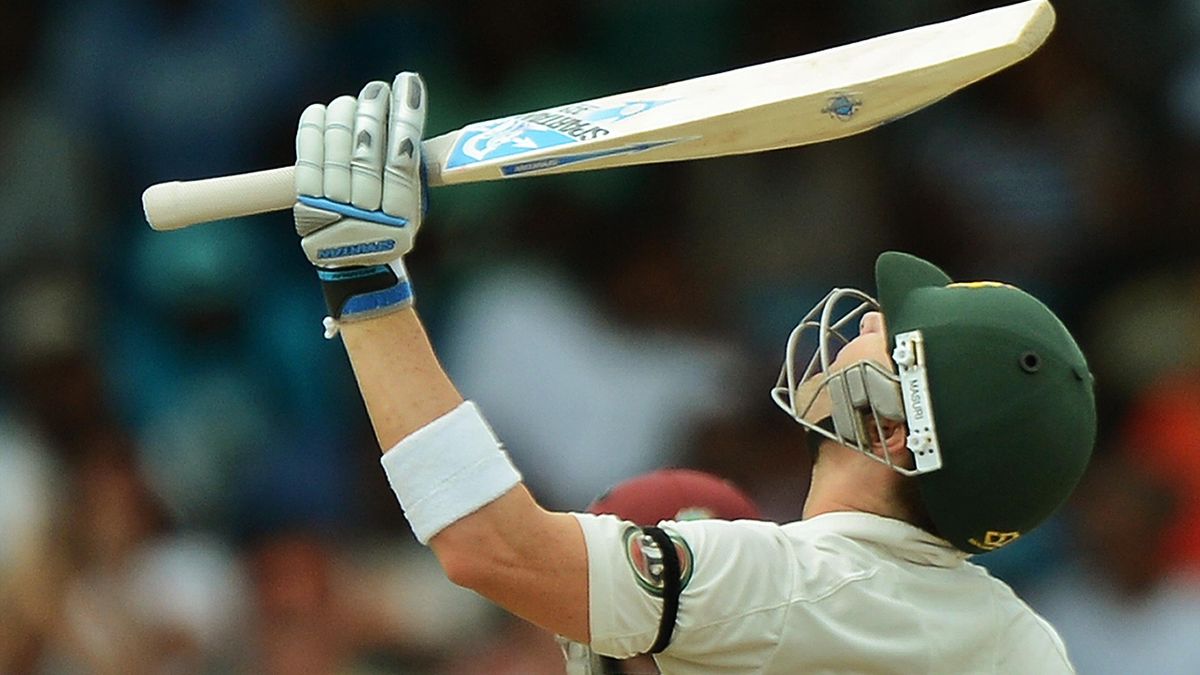In this high-definition photograph captured during a cricket test match, a Caucasian man is prominently featured, with his upper body clearly visible. He is adorned in a white or grey jersey, which has a black band on the sleeve above a logo to signify respect. The man wears a green helmet and is looking upwards, possibly in a moment of relief or triumph, suggesting he has just achieved a significant milestone such as a century or half-century. His left hand, adorned with a white band and grey gloves accented with turquoise and royal blue, is raised, gripping a beige cricket bat that has a blue side. The background is blurred, highlighting the audience in the stands and underscoring the focus on the player.